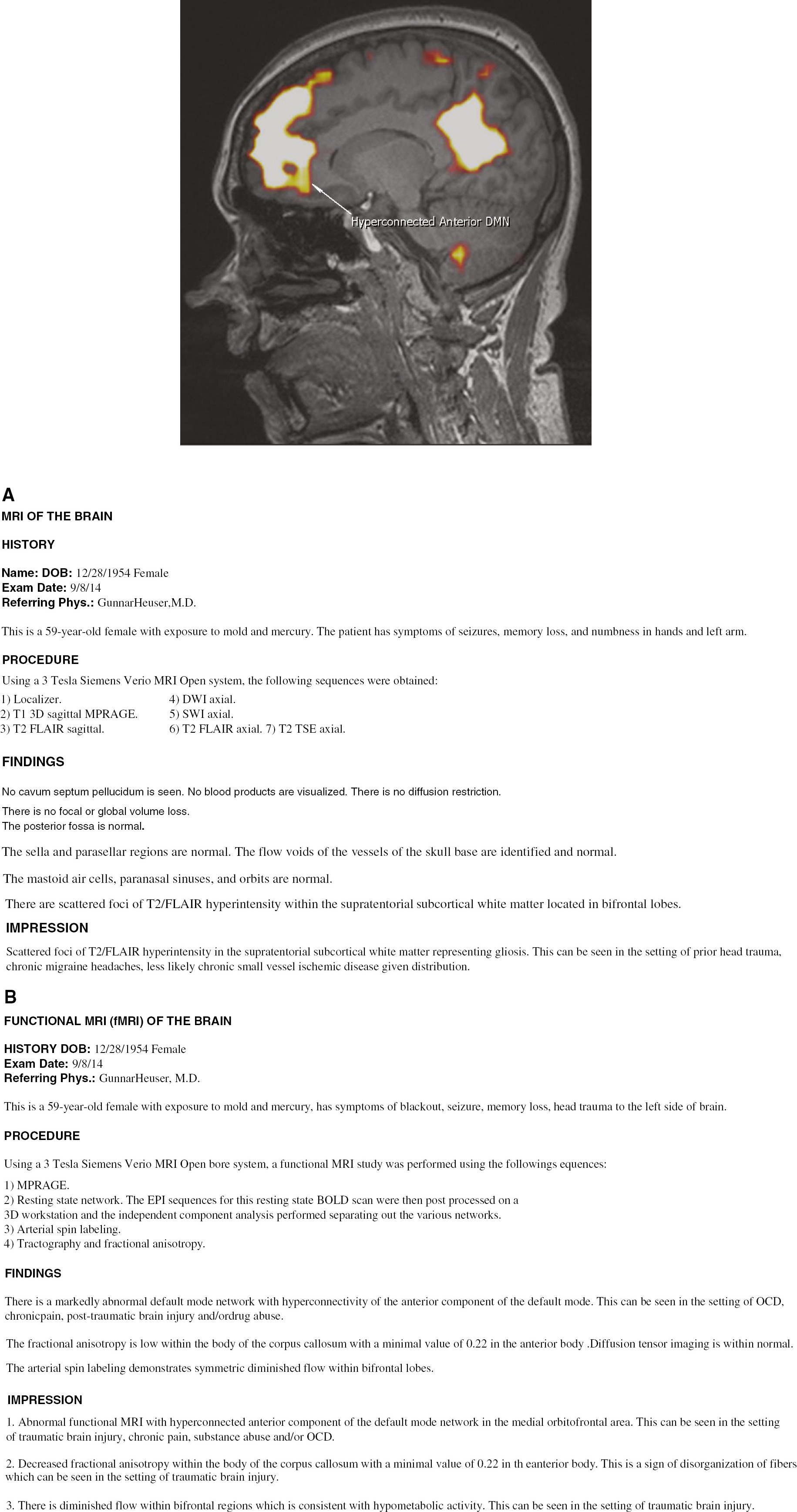The image shows a detailed medical document featuring an MRI scan of a patient's brain. The upper portion prominently displays the MRI image, capturing a side view of the head looking to the left. The brain is depicted in various shades of gray with specific regions highlighted in bright yellowish-white and outlined in dark red. Notably, the image highlights the anterior DMN with an arrow and a label in white text. Below the MRI image, the document includes detailed textual information such as the patient's date of birth (December 1954), gender (female), and summarized findings of the functional MRI (fMRI). This information is segmented into sections like history, procedure, findings, and impression, with the text indicating a hyperconnected anterior DMN. The document serves as a comprehensive report of the MRI findings, capturing both visual and textual data.